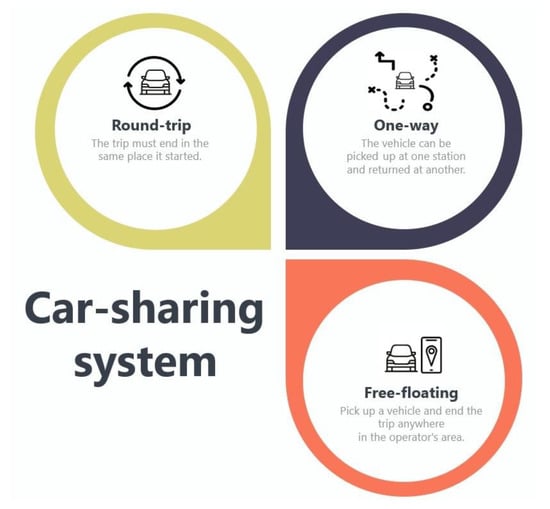The image is an informational sheet for a car-sharing system, featuring three different vehicle rental options, each color-coded and illustrated with icons. In the bottom left corner, "Car-Sharing System" is prominently displayed in blue text across two lines. The top-left quadrant is highlighted in a light olive green and labeled "Round Trip," specifying that the trip must end where it started. It includes a car icon surrounded by circular arrows. The top-right quadrant is marked with a navy blue color and titled "One Way," indicating that vehicles can be picked up at one station and returned to another. Illustrative arrows point in various directions with X marks at their endpoints. The bottom-right quadrant, colored orange, is labeled "Free-Floating," explaining that vehicles can be picked up and dropped off anywhere within the operator's area, accompanied by an icon of a car and a smartphone displaying a location icon. Each quadrant features a location icon with the pointed ends oriented towards the center, enhancing the visual organization of the information.